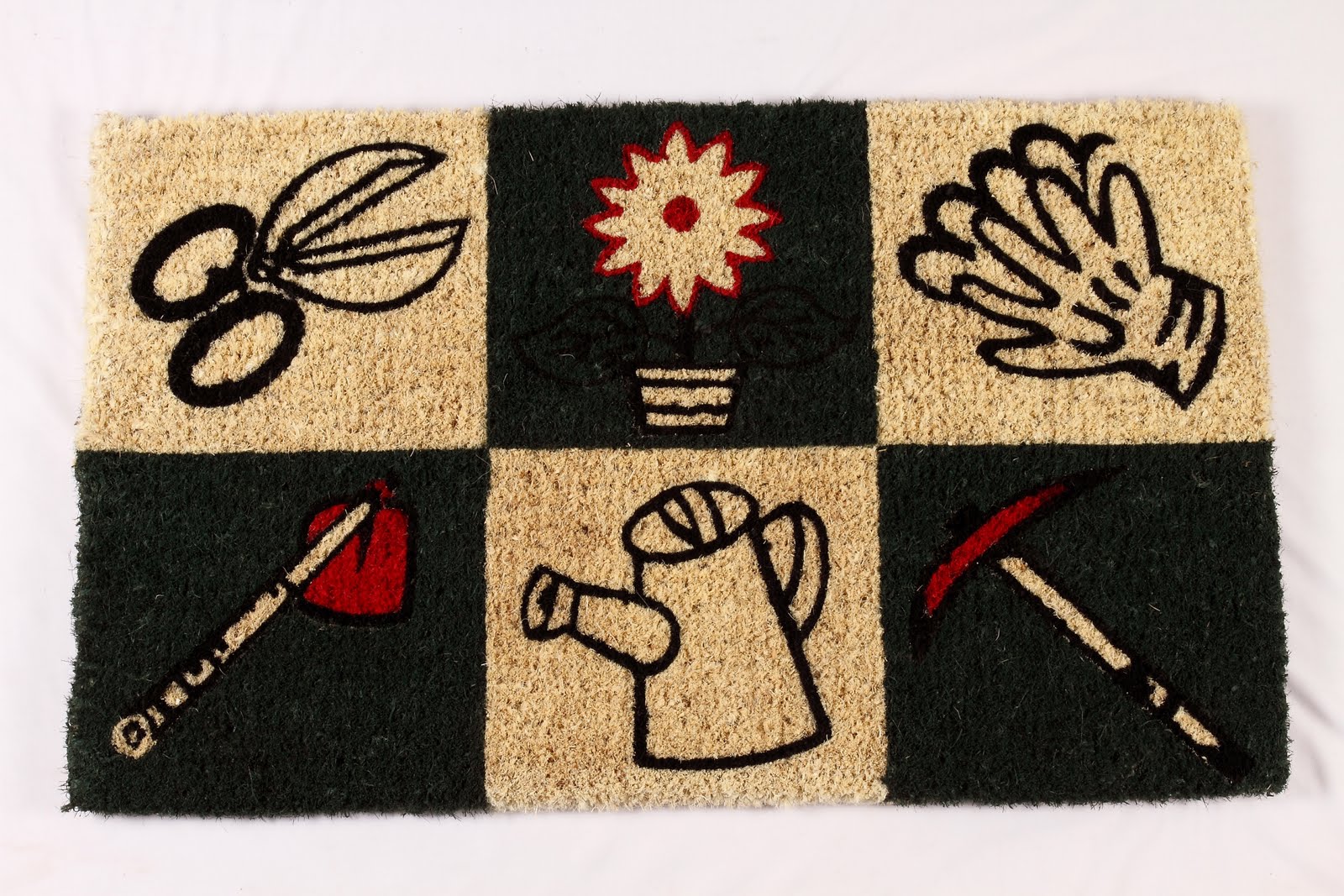This detailed image depicts a rectangular rug, likely utilized in a kitchen or as an outdoor mat for a front or back door. The rug is composed of alternating light beige and dark black squares, all framed by a white or off-white border. The top row features three squares: the leftmost square is beige with a pair of dark scissors angled to the right, the middle square is black with a red flower in a pot, and the rightmost square is beige with a pair of dark gloves. The bottom row also contains three squares: the left square is black with a garden hoe showcasing a red head and a beige handle, the middle square is beige with a dark watering bucket, and the right square is black with a tool that has a red tip and a beige handle, possibly resembling an umbrella or other garden implement. The overall impression suggests the rug is firm to the touch, contributing functionality alongside its vibrant and contrasting design elements.